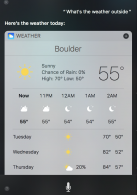This image captures a blurry screenshot of a weather app displayed on a cell phone. The overall background of the app is black, with various shades of grey used for different sections. 

At the top of the image, within a black header, there is right-justified text in the top right corner, though it's unreadable due to the blur. Below this header, a grey section contains left-justified text stating, "Here's the weather today."

Centered on the screen is a large, portrait-oriented grey block with rounded corners. The top line of this block is a slightly darker grey. On the left side, a blue square showcases an icon of the sun and a cloud. To the right of this icon, "WEATHER" is written in capital letters, and the top right corner features a close button represented by a circle with an X inside.

Within the next section of the grey block, the weather for the location "Boulder" is displayed in the center, marked by a thin grey line below it. The weather status is shown on the left with symbols and text. A bright sun icon indicates it’s sunny, with the text confirming "Sunny" and "Chance of rain 0%". The high and low temperatures are somewhat obscured but appear to read "High 70s, Low something." The current temperature reads 55 degrees.

Further down, another thin grey line separates this weather overview from the hourly forecast. The hours listed include 11 PM, 12 AM, 1 AM, and 2 AM, showing a forecast of "Partly Cloudy" for the later hours with corresponding moon icons. The temperatures for these times are listed as 55 degrees now, 65 at 11 PM, 64 at 12 AM, and 66 at 2 AM.

At the bottom of the grey block, another thin grey line precedes the daily forecast for Tuesday, Wednesday, and Thursday. For these days, the center column shows a sun icon for Tuesday and Wednesday, with a sun and cloud icon for Thursday, accompanied by a 20% chance of rain. Each day’s high and low temperatures are listed on the right-hand side.

The bottommost section of the image reverts to the black background, featuring a microphone symbol centrally positioned.